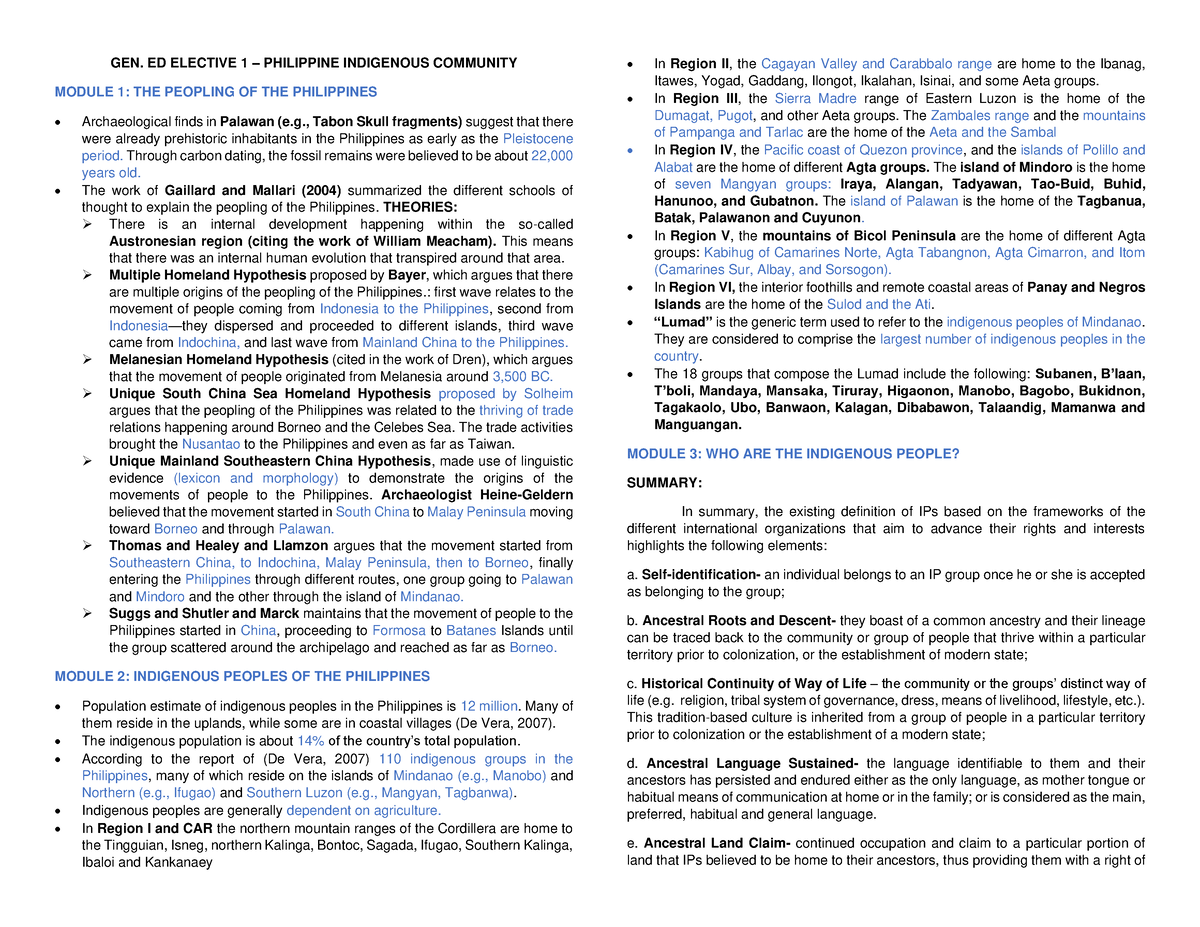Title: "Summary of Class Syllabus on Philippine Indigenous Communities"

Description: This image captures a summary of a class syllabus for the course "Gen.Ed Elective 1: Philippine Indigenous Community." The syllabus is laid out across two pages. 

- **Top Left Section:**
  - **Course Title:** In black text, it reads "Gen.Ed Elective 1: Philippine Indigenous Community."
  - **Module 1:** In blue text, the heading "Module 1: The People of the Philippines" introduces the first module.
    - **Main Bullet Points:**
      - "Archaeological Finds in Palawan."
      - "The Work of Gallard and Malari (2004)" followed by sub-bullet points with arrows:
        - Internal Developments in the Austronesian Region
        - Multiple Homeland Hypothesis
        - Melanesian Homeland Hypothesis
        - Unique South China Sea Homeland Hypothesis
        - Unique Mainland Southeast China Sea Hypothesis
        - Thomas & Healy and Lamazon Arguments
        - Suggs, Schulter, and Mark Arguments

- **Module 2:** In blue text, the heading "Module 2: Indigenous Peoples of the Philippines" introduces the second module.
  - **Main Bullet Points:**
    - Population Estimate and Indigenous Population Percentage (14%)
    - Number of Indigenous Groups: 110
    - Dependence on Agriculture
    - **Regional Breakdown:**
      - Region 1 and CAR
      - Region 2, covering the Ibang, Itaz, Yogart, Garang, Illinois, Ilkan, Isni, and Samayeta groups
      - Region 3: Sierra Madre region
      - Region 4: Quezon Province
      - Region 5: Bicol Peninsula
      - Region 6: Interior Foothills and Remote Coastal Areas
      - Lumad: Indigenous Peoples of Mindanao
      - The last 18 groups of the Lumad

- **Right Page Continuation:**
  - Extends the list of bullet points from the previous page.

- **Module 3:** In blue text, the heading "Module 3: Who Are the Indigenous People" introduces the third module.
  - **Summary Points:**
    - **A.** Self-identification
    - **B.** Ancestral Roots and Descent
    - **C.** Historical Continuity of Way of Life
    - **D.** Ancestral Language Sustained
    - **E.** Ancestral Land Claim